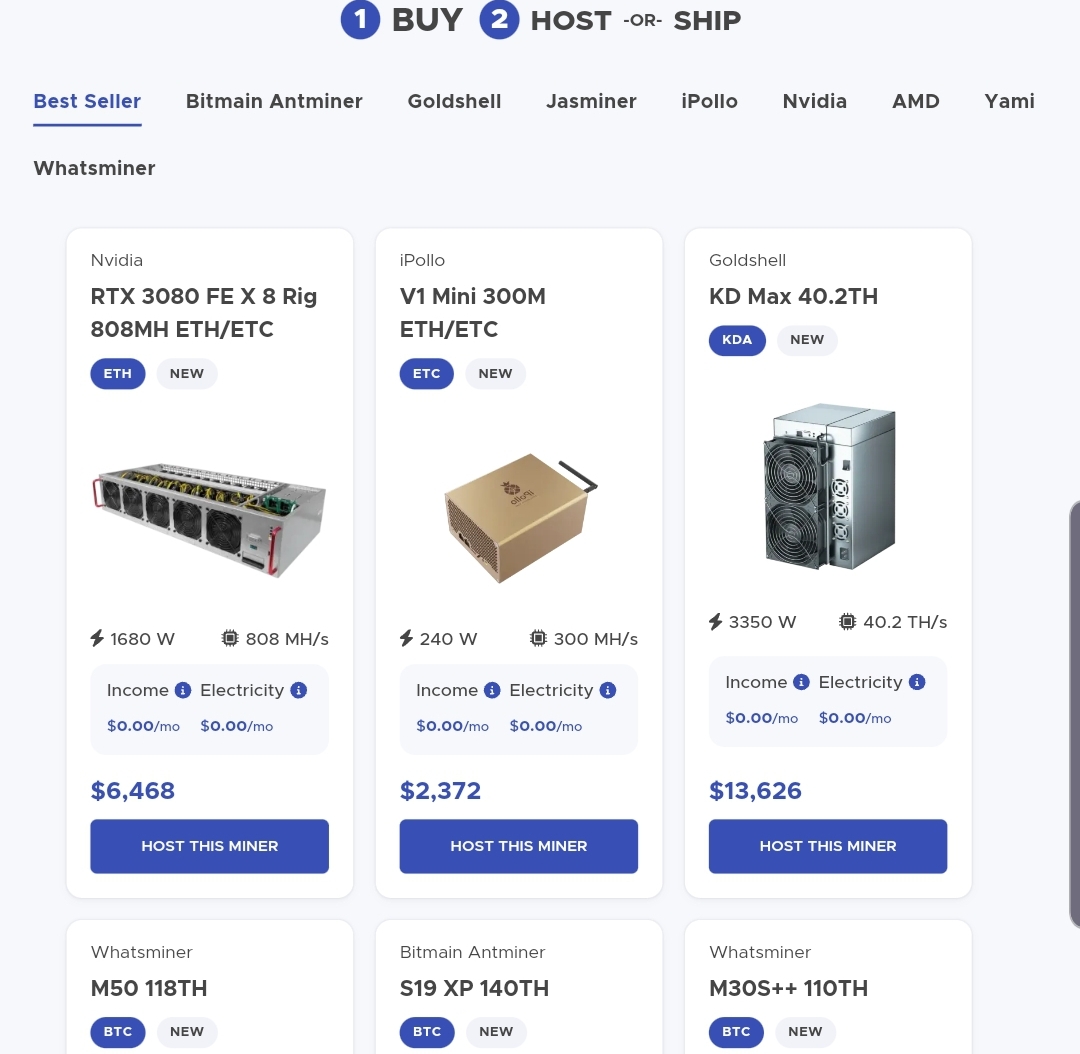This screenshot is from a website called "Buy, Host, or Ship," as displayed prominently at the top of the page. The navigation bar features three sections: "Buy" marked with a 1, "Host" marked with a 2, and "Ship" without any marking. The page comprises several tabs, with "Best Seller" being the currently active tab. Other tabs available include Bitmain, Antminer, Goldshell, Jazzminer, Apollo, NVIDIA, AMD, and YAMI.

Under the "Best Seller" tab, there is a category titled "What's Miner?" This section showcases various computer parts. The first item visible is an NVIDIA RTX 3080 FE X-Rig. Key specifications listed for this product are a wattage of 1680W and an operating efficiency of 808 mAh/s. The income and electricity cost for this miner are both noted as $0 per month. The product is priced at $6,468, and there is an option to "Host this Miner."

Other visible items include the Apollo V1 Mini 300M and the Goldshell KD Max 40.2 TH. Each product is accompanied by its respective image and brief specifications.